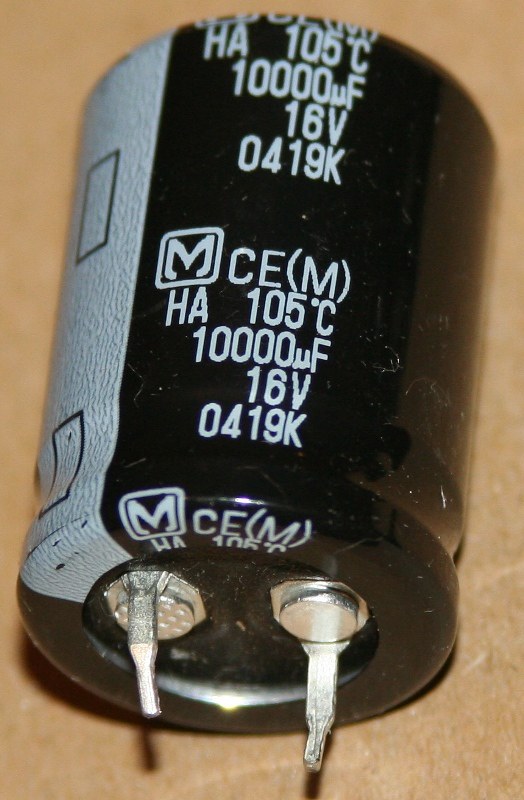The image depicts a close-up view of a black cylindrical capacitor, typically used in computer circuit boards and motherboards, against a tan background. The capacitor has a shiny, black outer casing with a vertically oriented white stripe along one side. The text on the capacitor reads "HA 105°C 10000µF 16V 0419K" in a whitish-gray color, with this information repeated further down on the device. The text includes a curved "M" logo, preceding the letters "CEM" in parentheses. At the bottom of the capacitor, two tiny metal legs protrude vertically downward, attached to silver brackets resembling bolts. Additionally, two rectangular shapes are visible within the vertical white stripe on the left side. The capacitor's surrounding surface appears to be shrink-wrapped in a shiny plastic material.